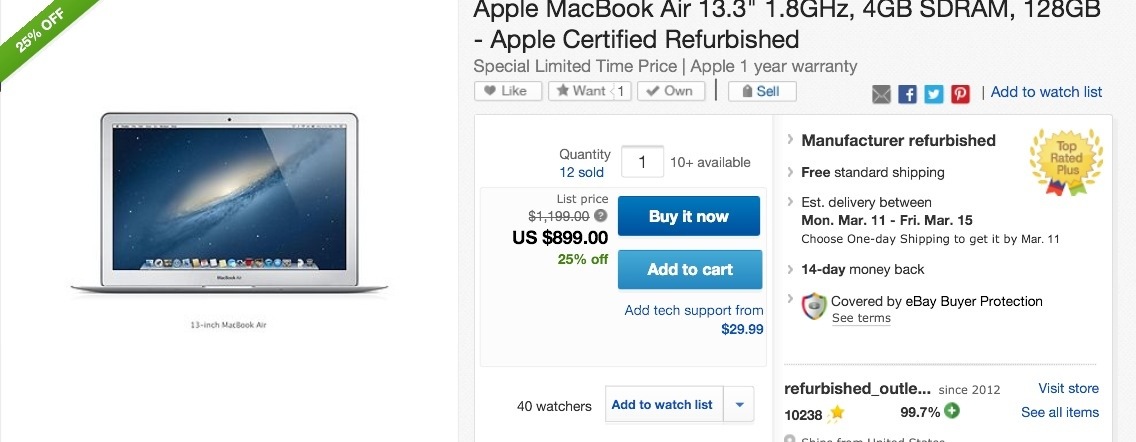The image features a clean white background and appears to be a screenshot from an e-commerce website, likely showcasing an advertisement. The ad is for an Apple MacBook, specifically the MacBook Air model. The visual of the laptop on the left side is not a real photograph but a digital drawing. Prominently displayed on this image is a green ribbon with "25% off" written in white, located at the top of the box containing the MacBook graphic.

The layout of the ad is rectangular, with approximately one-third dedicated to the MacBook image and the remaining space used for descriptive text. The text details the product as an Apple MacBook Air with a 13.3-inch screen, a 1.8 GHz processor, 8 GB of SDRAM, and a 128 GB SSD. It is clearly labeled as Apple certified and refurbished.

Below the product description, there are interactive buttons for social engagement including options to like it, want it, own it, or sell it, accompanied by various social media icons. These buttons stretch across the area beneath the product's name. 

The ad indicates there are over 10 units available and features two central action buttons: one blue "Buy It" button and a slightly lighter blue "Add to Cart" button. On the far right side, additional product information is displayed, noting that it's manufacturer refurbished, offers free standard shipping, and includes a "Top Rated Plus" gold ribbon for added emphasis on quality and reliability.